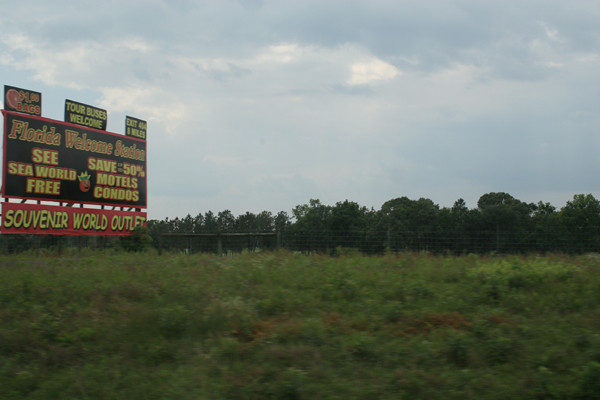In this somber, dimly-lit daytime scene, a dreary field stretches out before us. The grass is uneven and scrubby, indicating perhaps a lack of maintenance or the harsh effects of seasonal weather. Dominating the left side of the landscape is a vibrant billboard adorned in bold red, black, and yellow colors. The bottom red band of the billboard prominently advertises “Souvenir World Outlet.” Above, the central portion of the billboard warmly welcomes travelers with the announcement “Florida Welcome Station.” It also entices visitors with promotional messages such as “See SeaWorld Free,” and “Save up to 50% motels condos,” highlighting potential savings and attractions. The billboard is further adorned with smaller, auxiliary signs that stick out from its top. Directly ahead in the scene, a barbed wire fence reinforced with wooden posts and supports runs horizontally across the field, creating a boundary. Beyond the fence, a line of tall trees looms in the distance, their presence adding a sense of depth and isolation to the overall mood of the landscape.